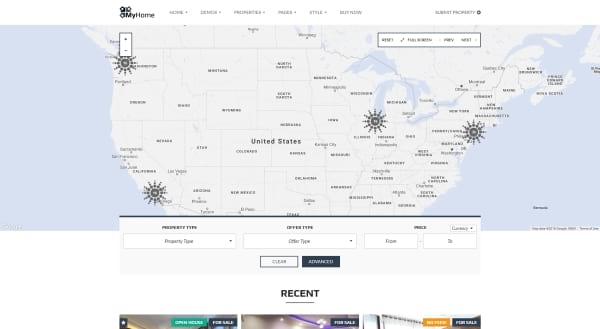This image appears to be a screenshot of a website page, likely a property or real estate platform. The page header in the top-left corner displays the title "My Home" in black. Although the header contains tabs, only the "Style" tab is slightly visible, with the others obscured.

At the center of the page, there is a detailed world map highlighting the United States. Surrounding the map are oceanic expanses to the left and right. Specific cities and countries are marked, with notable black solid circles indicating key locations (two on the right side of the map and two on the left side).

Towards the bottom of the map, there are several interactive elements. Users can find drop-down menus allowing selections for property type, offer type, and date ranges (from and to). Below these menus, two buttons are positioned: a gray "Clear" button with white text, and a black button with text that is not clearly visible. However, beneath this button, the label "Recent" is displayed.

The lower section of the image also showcases three static horizontal pictures, providing visual content related to the website's offerings.